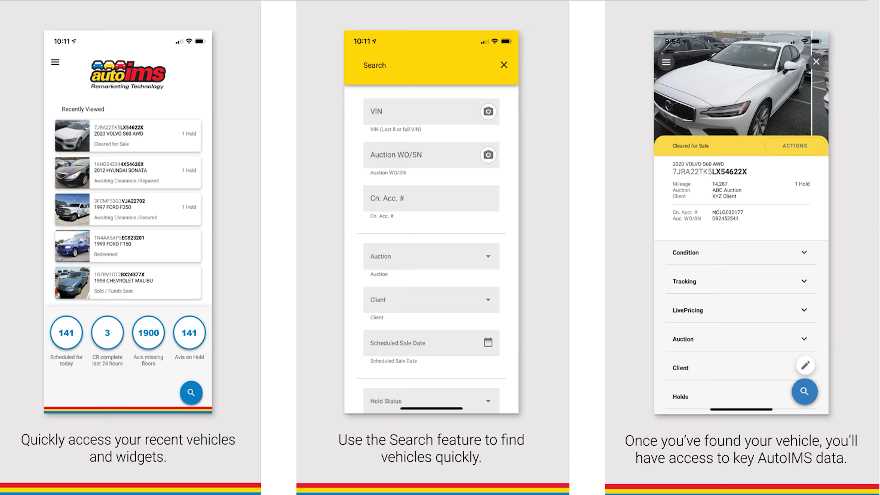The image features three smartphone screens displayed side by side, each depicting content related to automobiles. The screens appear to be showcasing a car dealership or automotive inventory management application.

**Left Screen:**
This screen displays a grid of five cars, each accompanied by photos and some text offering details about these vehicles. However, the image resolution is poor, making the information difficult to read. Beneath the car listings, there are four blue circles outlined in white, each containing a number. From left to right, the numbers are 141, 3, 1900, and 141. Below these numbers, there is a text section titled "Quick Access," which provides shortcuts to recently viewed vehicles and widgets.

**Middle Screen:**
The central screen features a search bar, encouraging users to "use the search feature to find vehicles quickly." This section likely serves as the main interface for users to input queries and locate specific cars within the inventory.

**Right Screen:**
The rightmost screen highlights a single vehicle, a white coupe. Below the image of the car, text indicates that once a vehicle is found, users will have access to essential Auto IMS data. This section appears to be tailored for detailed vehicle information once a specific car is selected.

**Background:**
The three smartphone screens are set against a gray background, enhancing their visibility and separating them from any other visual elements.

Overall, the image provides a glimpse into a user-friendly application designed to facilitate quick access to car information.